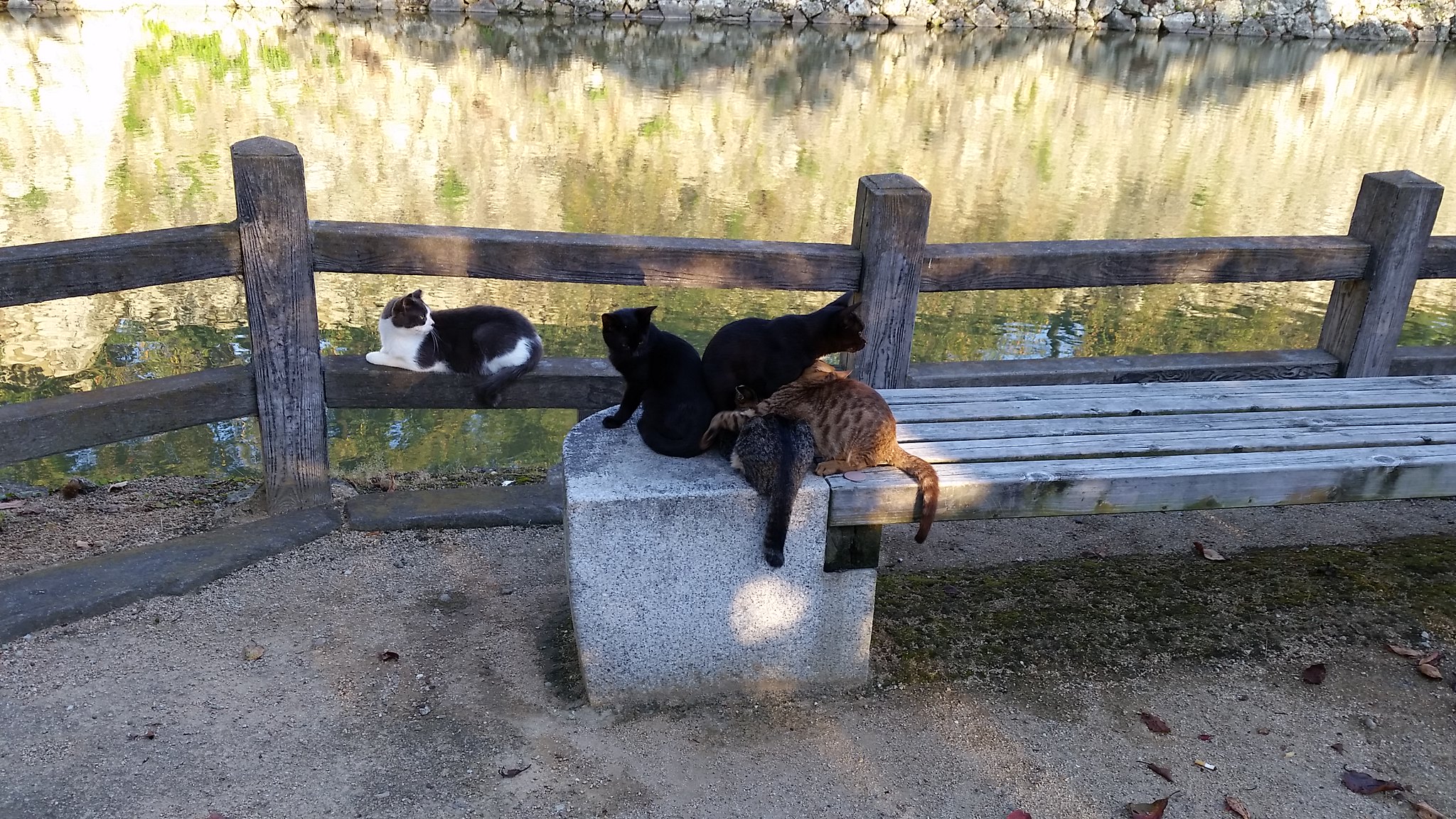The photograph captures an outdoor scene with a detailed setting and focal points. In the foreground is a large concrete block attached to several long, deep wooden boards forming a bench. The center section of the photograph prominently displays this bench, which hosts four distinct cats: two black cats, one brown tabby, and one mottled gray tabby. Each cat sits in various poses, with the tabbies facing upward, one black cat looking downward, and the other gazing rightward. Immediately behind the bench, a wooden fence features three horizontal beams and square wooden posts. On the middle beam of this fence sits a black-and-white tuxedo cat, positioned slightly to the left and looking right. Beyond the fence, a grassy area with slightly faded tall brown grass leads to a waterway whose surface reflects distorted foliage, likely stemming from off-camera trees. At the very top of the image, a stone wall completes the backdrop, contributing to the overall serene and rustic ambiance of the scene.